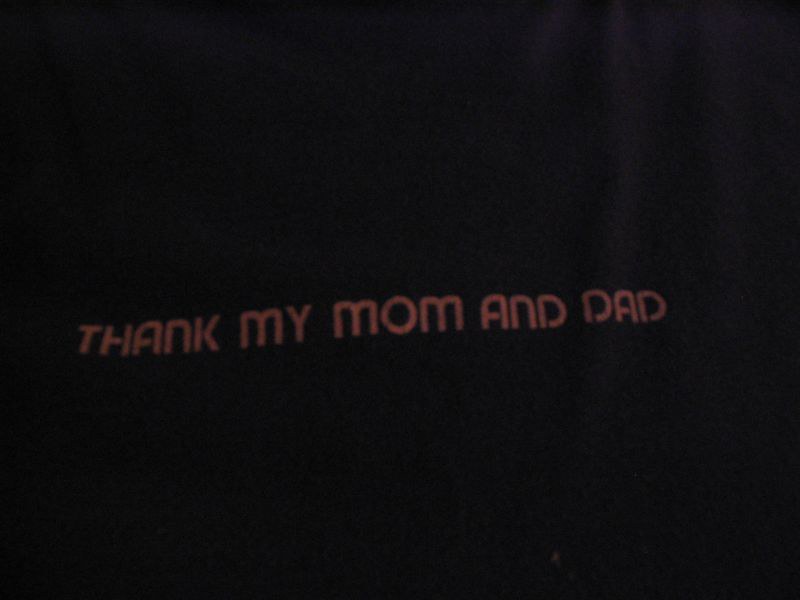The image displays a solid black background with uppercase red text in a curvy font. The text reads "THANK MY MOM AND DAD." Each letter is distinct, and the font style leaves small gaps, particularly noticeable in the letters H, A, N, and D. The stark contrast between the vivid red lettering and the deep black background draws immediate attention to the message, which appears both bold and heartfelt.